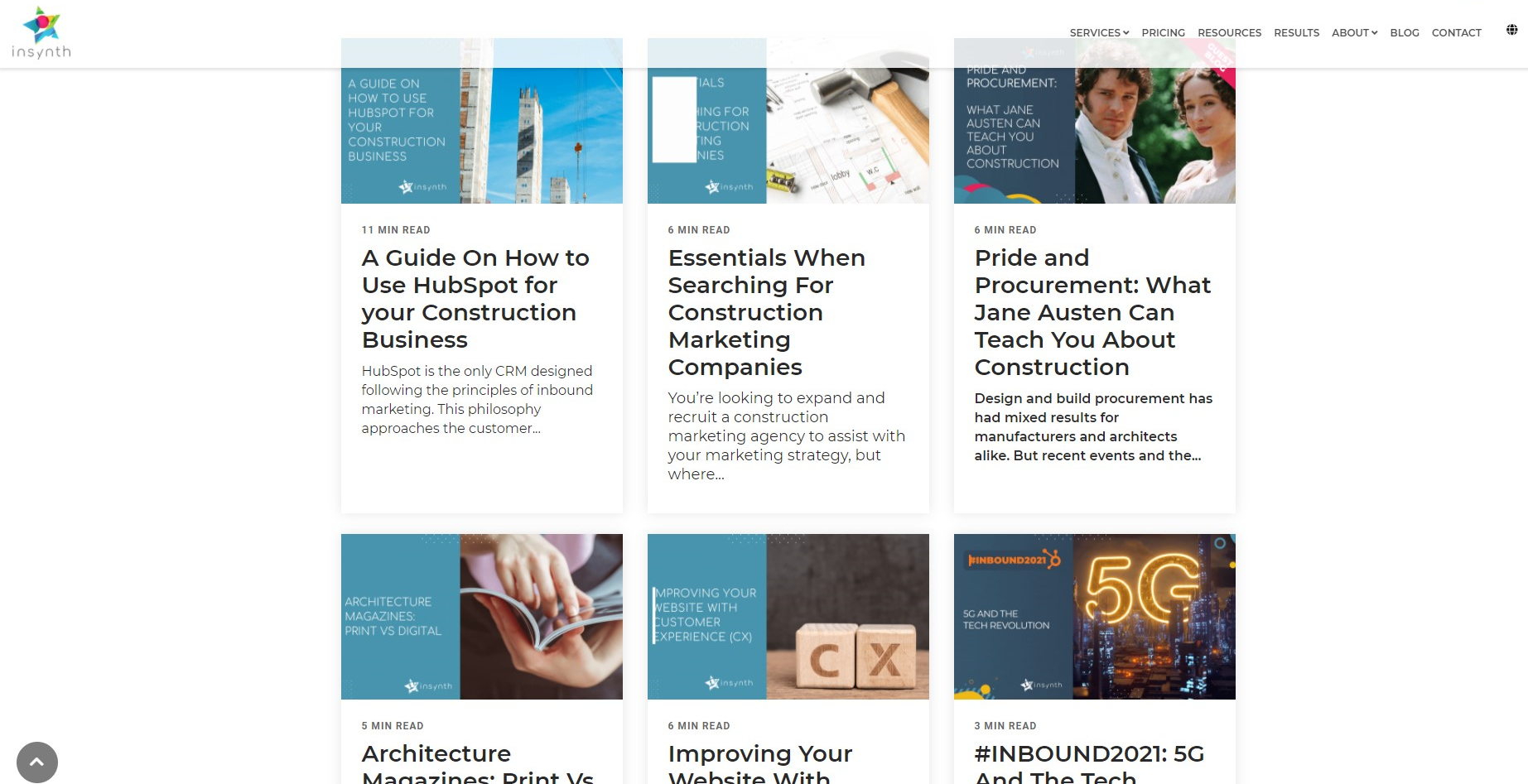This detailed caption provides an in-depth description of the contents and layout of the screenshot image:

The image is a screenshot of a website. In the top left corner, there is a multi-colored star graphic. Below the star, in lowercase letters, is the word "INSYNTH." Located at the top right of the image, there's a horizontal menu with the following options: Services, Pricing, Resources, Results, About, Blog, and Contact. 

Beneath this menu bar, several article titles and brief descriptions are listed, each followed by the estimated reading time:

1. "A guide on how to use HubSpot for your construction business. 11-minute read. HubSpot is the only CRM designed following the principles of inbound marketing. This philosophy approaches the customer..."
2. "Essentials when searching for construction marketing companies. Six-minute read. You're looking to expand and recruit a construction marketing agency to assist with your marketing strategy, but where..."
3. "Pride and Procurement: What Jane Austen can teach you about construction. Six-minute read. Design and Build Procurement has had mixed results for manufacturers and architects alike, but recent events and the..."
4. "Architecture magazines: print versus digital. Six-minute read."
5. "Improving your website with customer experience (CX). Three-minute read."
6. "Hashtag Inbound 2021: 5G and the tech revolution."

The image itself is wider than it is tall, showcasing the website's layout and featured contents clearly.